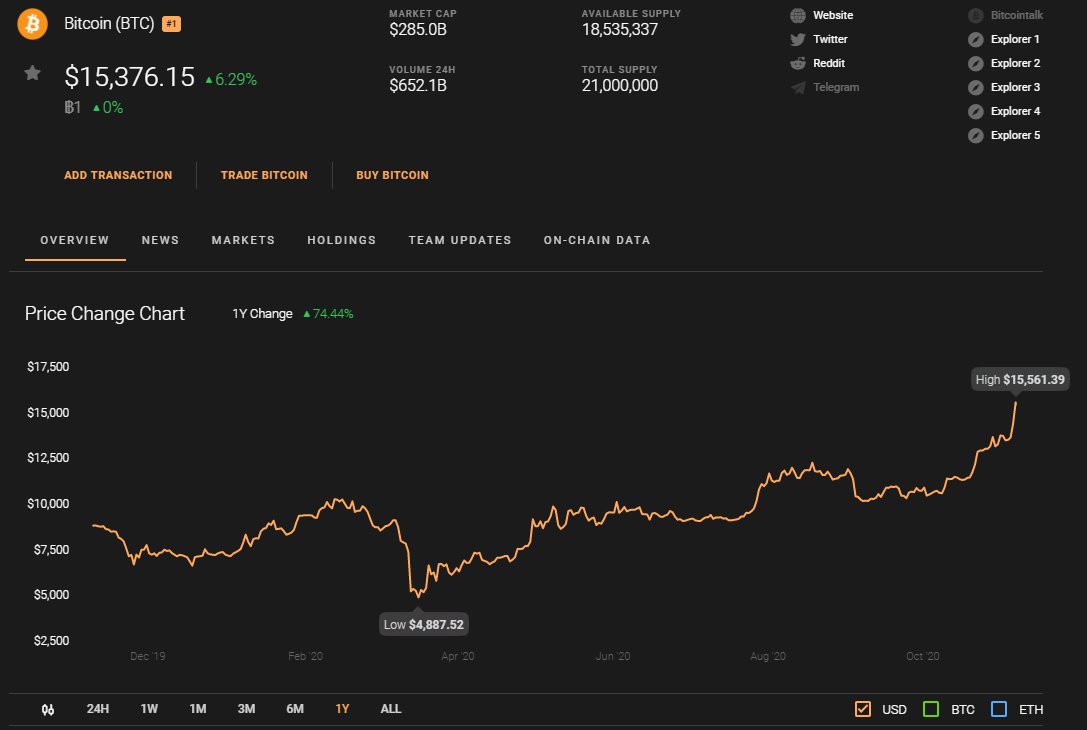A detailed screenshot depicts a Bitcoin stock interface dominated by a black background with white text. In the top-left corner, an orange circle features a prominent white "V". Adjacent to the icon, "Bitcoin (BTC)" is clearly labeled, along with an additional small orange button beside it. Below this section, there's a gray star followed by the numbers "15,376.15". Beneath the numbers, a green "+6.29%" is displayed indicating a positive change. The sequence continues with "B1" in white text, accompanied by a green upward arrow showing "0%".

To the right of these indicators, a column of various numerical data is presented in white text, which likely corresponds to different stock metrics. Directly below this text column are three horizontal orange tabs. Positioned beneath these tabs are six clickable white tabs offering more options.

Lower on the interface, a "Price Change Chart" section showcases a fluctuating line graph indicating Bitcoin price changes over time. The graph features an orange line that visibly trends upward amidst its zigzag pattern. Dates are labeled along the bottom axis of the graph. Finally, in the bottom-right corner of the screenshot, there are three distinguishable colored squares, each of a different hue.